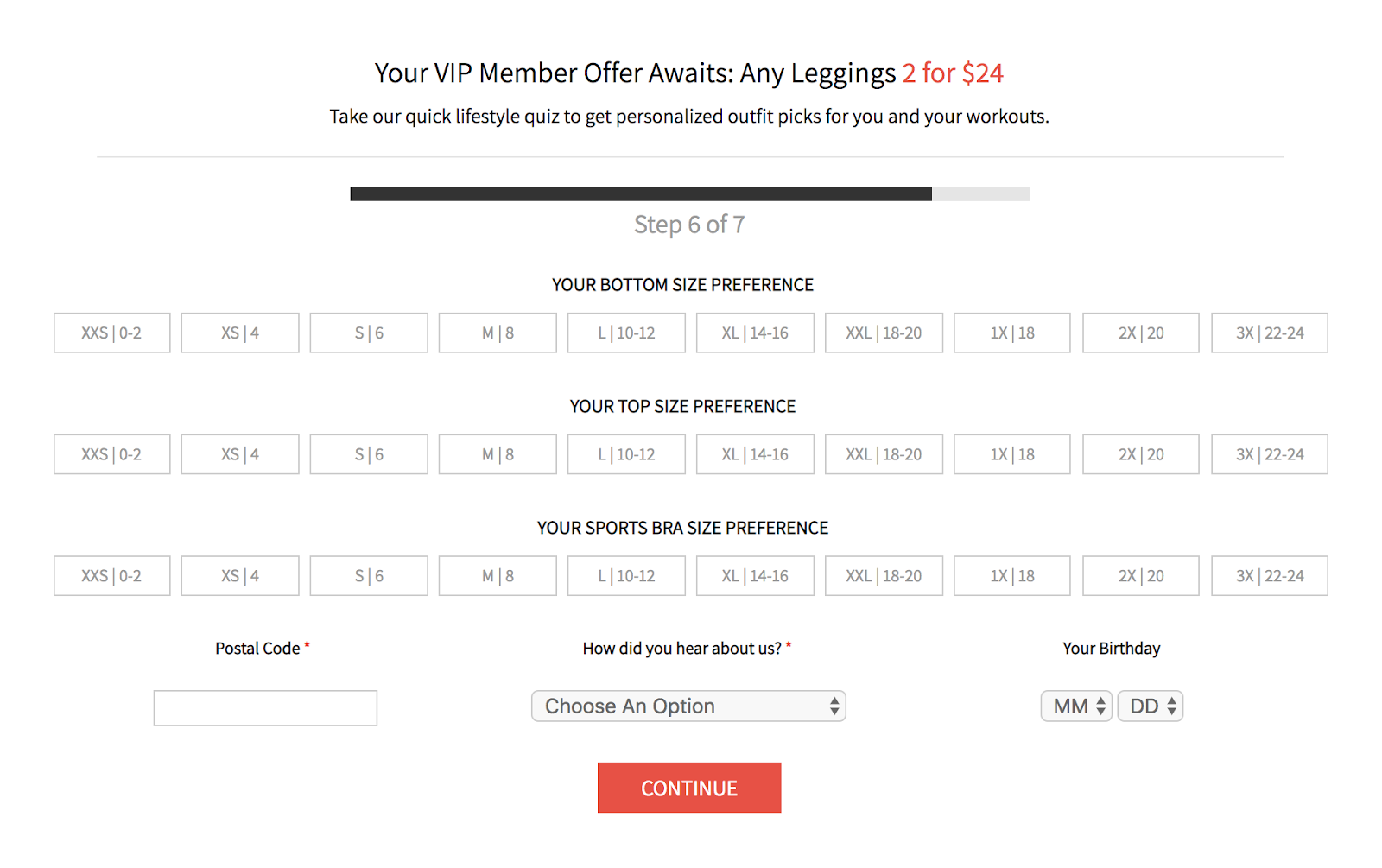"Unlock Your VIP Offer: Complete Our Lifestyle Quiz for Personalized Activewear at $24 Per Item! 

Take the quick lifestyle quiz to receive tailored outfit suggestions based on your workout preferences and style. 

### Step 6-7: Choose Your Sizes 
#### Bottom Size:
- XXS (0-2)
- XS (4)
- S (6)
- M (8)
- L (10-12)
- XL (14-16)
- XXL (18-20)
- 1X (18)
- 2X (20)
- 3X (22-24)

#### Top Size:
- XXS 
- XS 
- S 
- M 
- L 
- XL 
- XXL 
- X 
- 1X 
- 2X 
- 3X 

#### Sports Bra Size:
- XXS 
- XS 
- S 
- M 
- L 
- XL 
- XXL 
- LX 
- 2X 
- 3X 

### Final Steps:
1. Enter your postal code (mandatory).
2. Let us know how you heard about us (required).
3. Provide your birthday (MM/DD format).

Click 'Continue' to finalize your participation and discover your exclusive deals!"